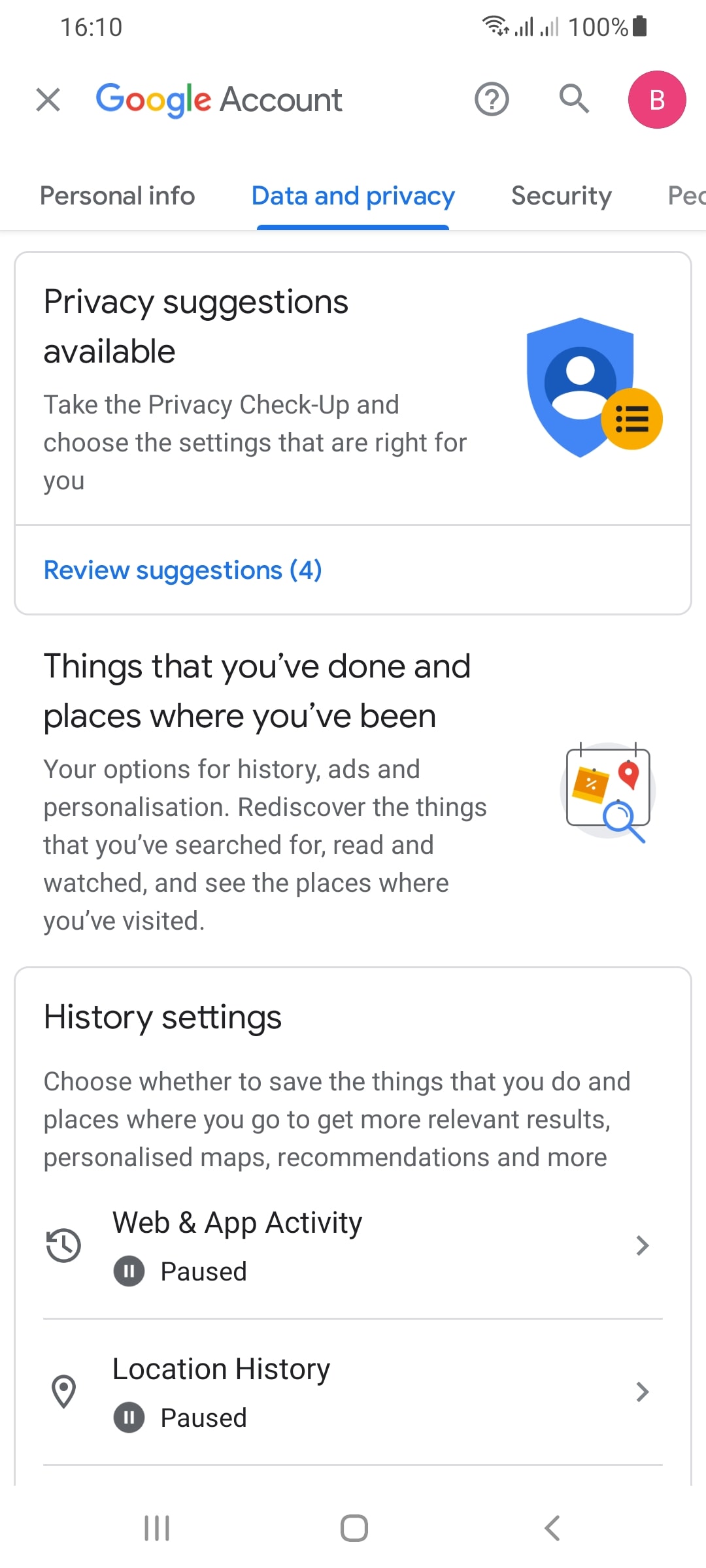The image depicts a Google account interface on a mobile phone. The time displayed at the top of the screen is 16:10, and the battery is fully charged at 100%. Below this, the familiar, multicolored Google logo is prominently featured, accompanied by search and user icons.

The main section of the screen offers various options related to personal information, data privacy, and security. The user has selected the 'Data & privacy' section, which reveals further details. Here, there is a box titled "Privacy suggestions available," prompting the user to review four suggestions, such as taking the Privacy Checkup to choose settings that suit their needs.

Further down, a section labeled "Things you've done and places you've been" provides options to manage history, ads, and personalization. It encourages the user to rediscover their searches, readings, and watched content, as well as to review visited places. Another box, titled "History settings," invites the user to decide whether to save their activity and location data to receive more relevant results, personalized maps, and recommendations.

Despite these prompts, the user's 'Web & App Activity' and 'Location History' settings are both shown as paused.